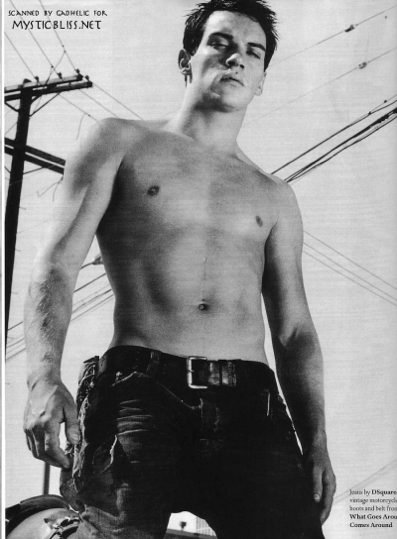The black-and-white scanned image from a magazine features a striking fashion photograph of a shirtless man standing in the center of the page, against a stark sky backdrop crisscrossed by utility lines and poles. The man, who has short, dark hair and no chest hair, is depicted wearing blue jeans secured with a prominent black leather belt and buckle. His demeanor is intense, with a downward gaze towards the camera; his eyes are partially closed, and his mouth remains shut, giving an impression of discomfort or annoyance. The photograph taken from a low angle accentuates his imposing presence, reminiscent of Michelangelo's David. At the top left of the page, there's text reading "scanned by Gadhill for mysticbliss.net," while tiny text at the bottom right reads "Jeans by D Square."